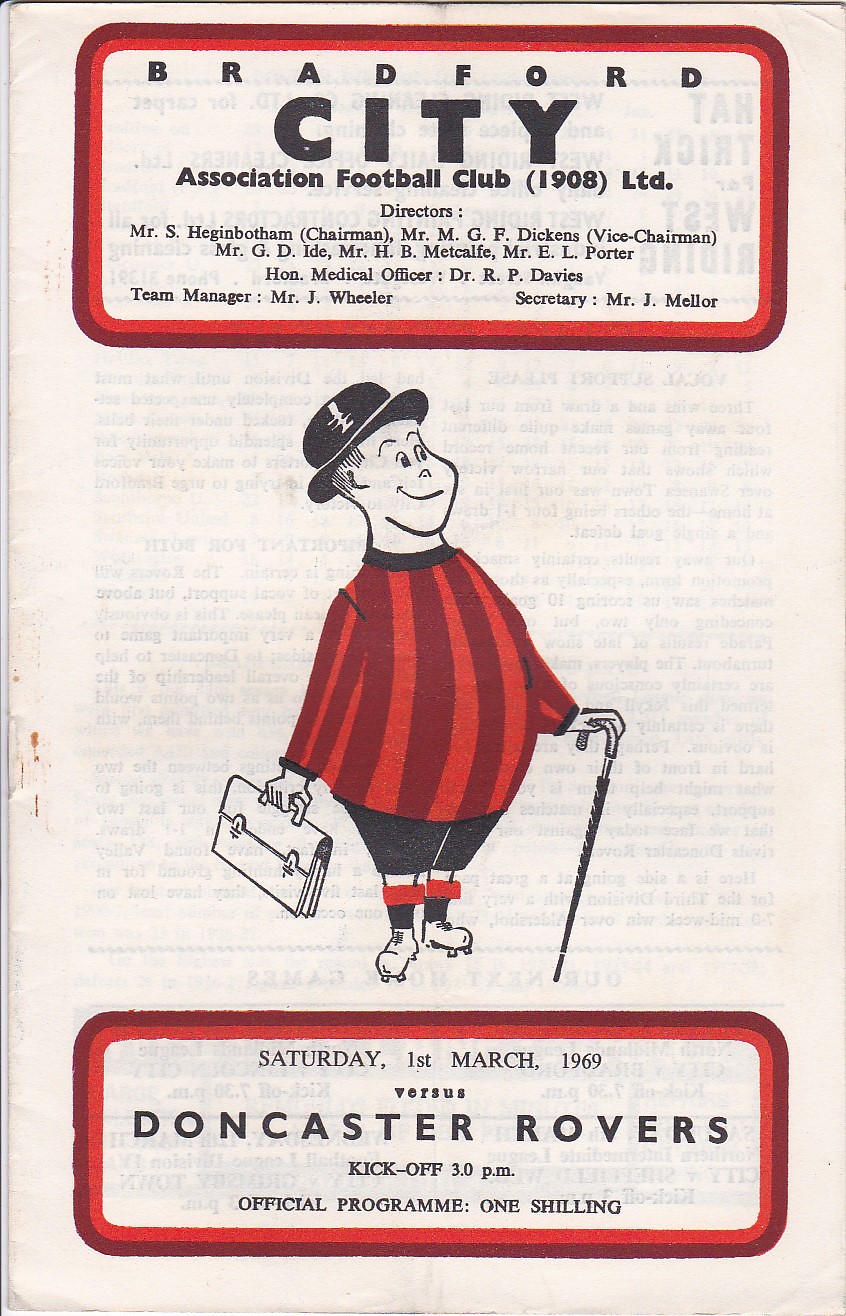The image depicts an aged front cover of an official program booklet for a soccer match dated Saturday, 1st of March 1969, between Bradford City Association Football Club (1908 Ltd) and Doncaster Rovers. At the top, within a box with a dark red outer line and a bright red inner line, the title reads "Bradford City Association Football Club 1908 Ltd" in black font, with "City" prominently in large, all caps letters. Below this title, the booklet lists information about the club's directors, including names like Mr. S. Hagenbotham, Chairman, and Mr. G.F. Dickens, among others.

Dominating the center of the cover is an illustrated figure reminiscent of a Monopoly character, wearing a red and dark red striped long-sleeve shirt, black top hat, and soccer cleats. The figure is smiling, holding an umbrella in one hand and a briefcase in the other. His attire features alternating dark raspberry and bright maroon vertical stripes. 

Below the figure, another box with a red border contains details of the match: "Saturday, 1st of March 1969 versus Doncaster Rovers, kickoff 3 p.m," with the program priced at one shilling. The transparency of the aged paper allows some text from the next page to show through.